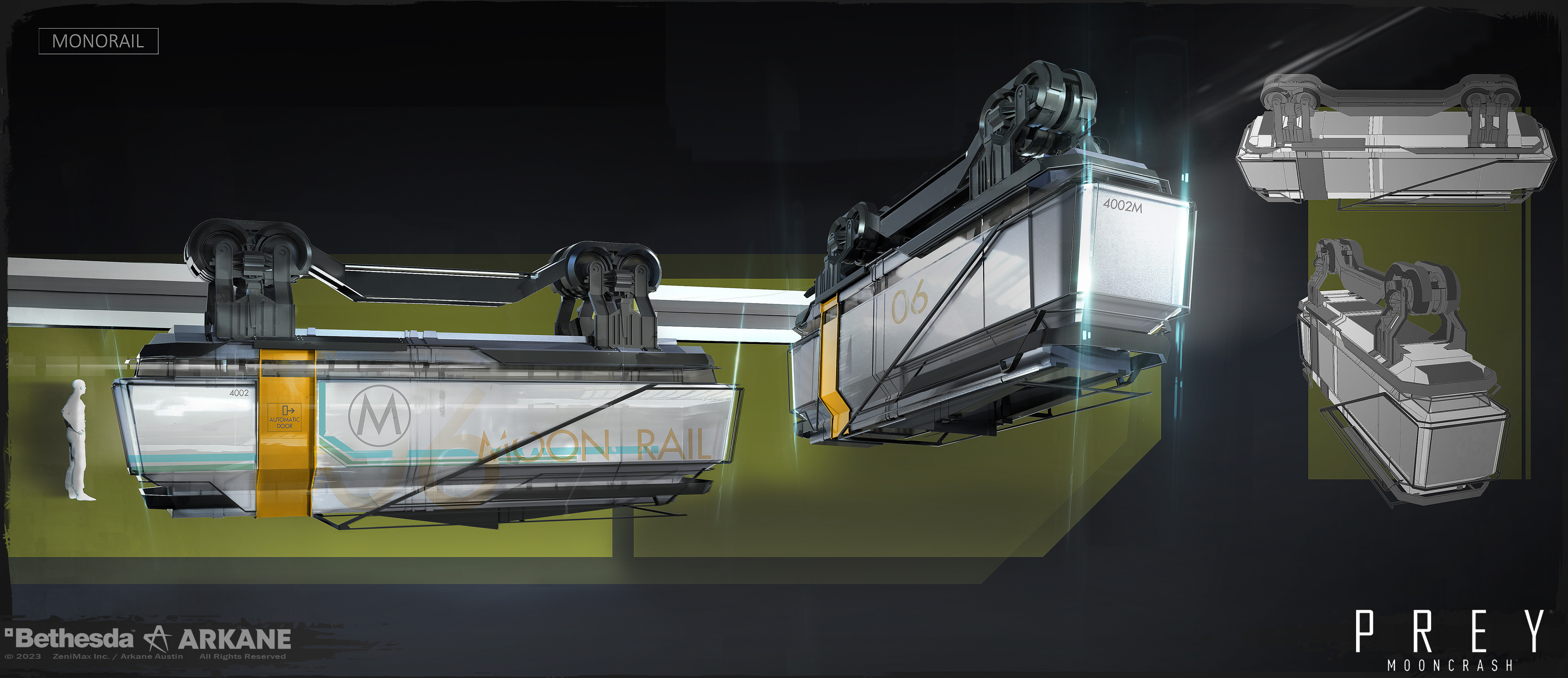The creative multi-color digital artwork depicts a horizontally rectangular scene set against a black background without a border. Prominently, in the lower right-hand corner is the word "PREY," followed by smaller lettering "MOONCRASH." The bottom left-hand corner features the text "BETHESDA ARKANE." The main focus of the image is a futuristic monorail system named "MOONRAIL," featuring vehicles that hang from a top-running track. The monorail cars, showcased from different angles, resemble upside-down train cars or gondola systems, with glass-sided structures. For scale, a small, white human figure is included on the left side, casting a faint shadow to emphasize the size contrast between the person and the monorail system. The overall background is speckled with dark green shapes, adding depth and complexity to the composition, while the monorail cars and person create an interesting and dynamic visual contrast.